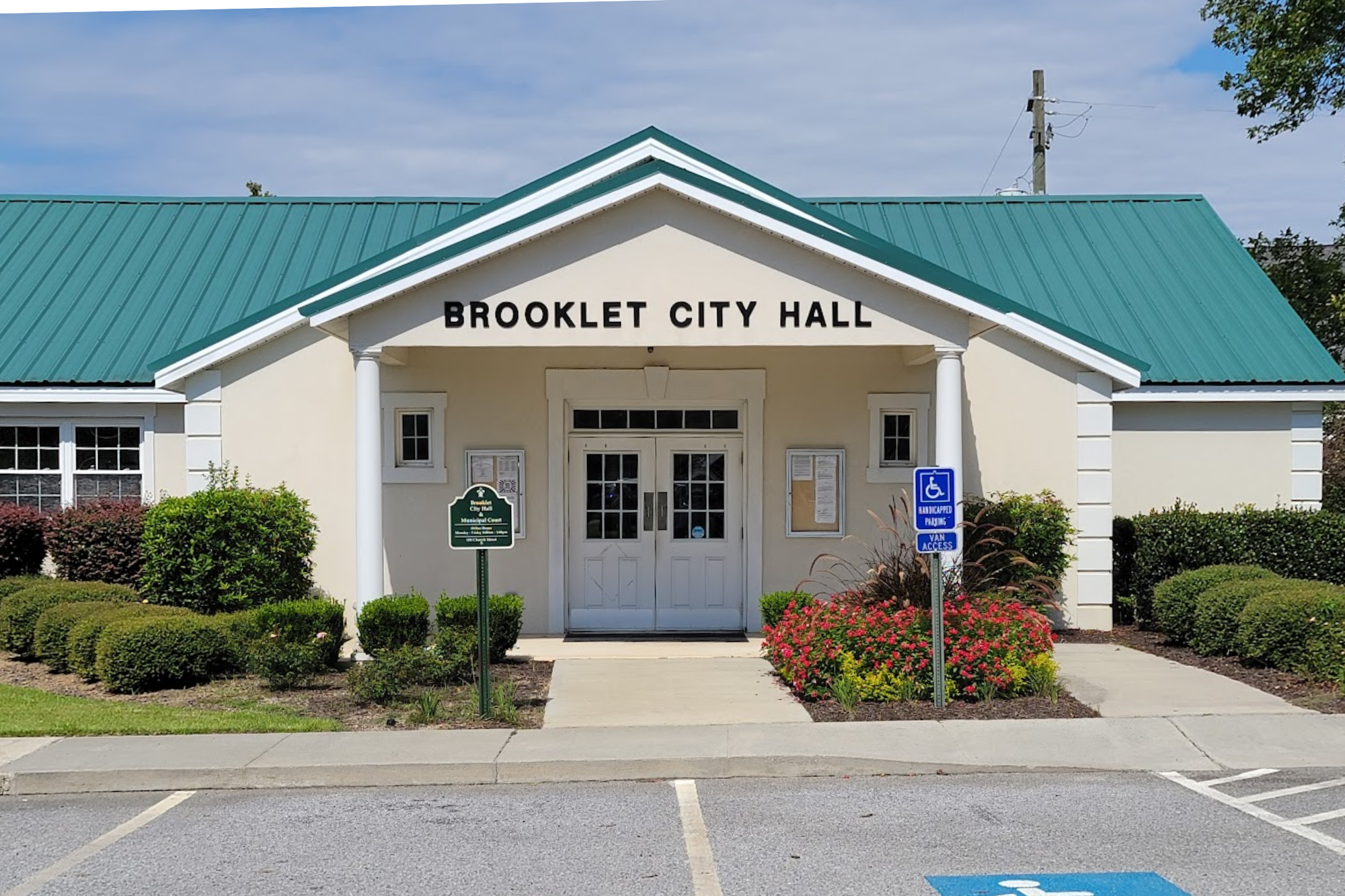This photograph showcases the front of Brooklet City Hall, a one-story building with a distinctive green metal roof and a cream-colored facade adorned with white stone pillars. Above the entrance, black capital letters spell out "Brooklet City Hall." The building features double white doors with glass windows, shaded by a roof overhang. 

In front of the entrance, there are well-maintained green bushes, as well as some red-hued bushes and flowers with red petals near the columns supporting the overhang. The view includes a portion of a light gray parking lot with three parking spaces, including one handicapped spot marked by a blue sign indicating van access.

A mix of green grass and additional bushes can be seen on the left side, along with a square-shaped green sign with a rounded top, the text of which is unclear. The backdrop reveals a blue sky populated with white clouds, indicating a sunny day that adds to the vibrant atmosphere of the scene. The overall composition clearly depicts the community-focused and accessible nature of the Brooklet City Hall.